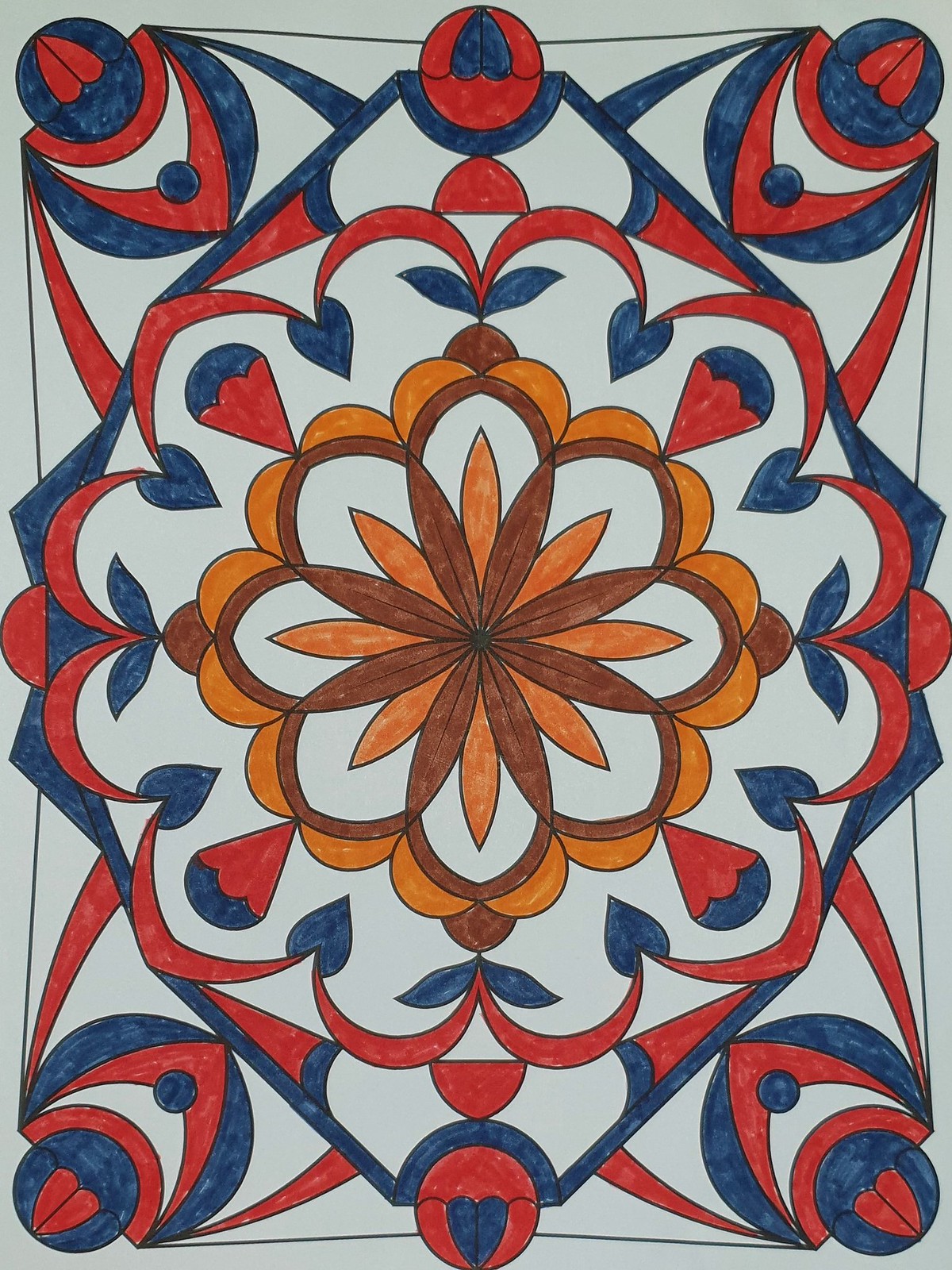This detailed caption emphasizes the key elements of the image:

"This photograph captures a page adorned with crayon or possibly watercolor art, characterized by a slightly gray backdrop. The predominant feature is a flower centered within the page, reminiscent of a mandala but set within a rectangular frame. The flower itself is vibrantly colored in shades of brown and orange. Surrounding the flower are intricate leaves and scroll-like patterns in red and blue, extending outwards to meet similarly hued designs in the corners. The coloring appears to be applied with a casual, unrefined technique, showcasing visible crayon marks or uneven watercolor strokes, suggesting the artwork was created for the artist's personal enjoyment."